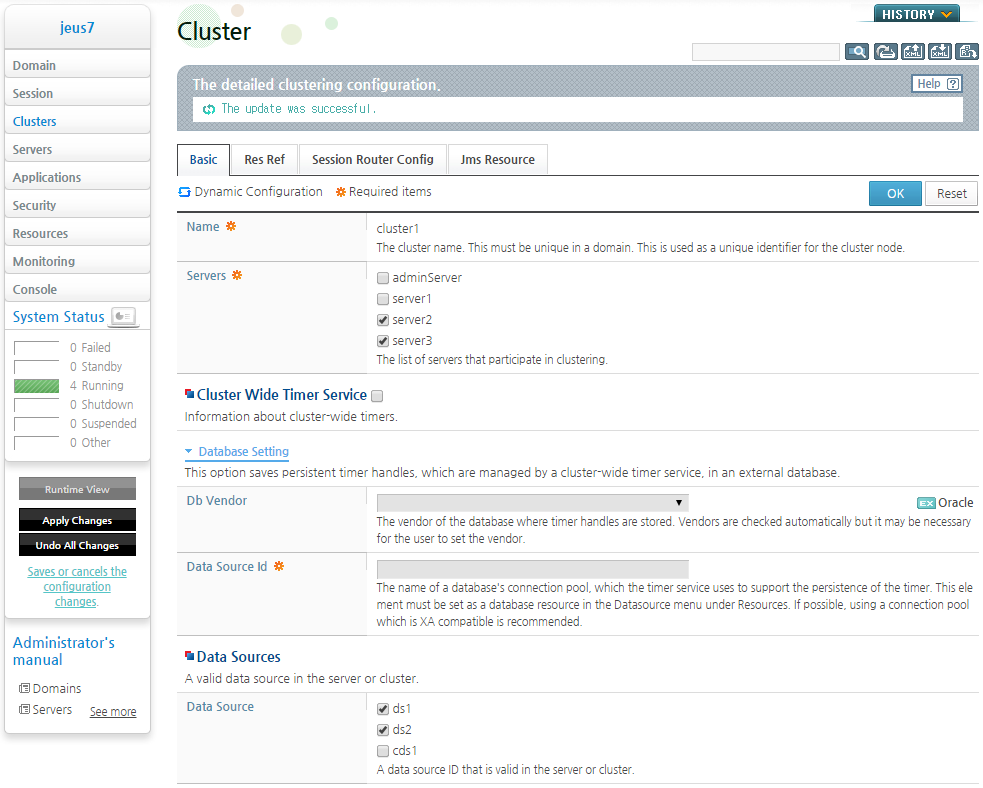The image depicts a detailed interface of a software management console. On the left side, the heading "G-E-U-S 7" is prominently displayed. Below this, a series of blue-highlighted options are listed, including "Domain," "Session," and "Clusters." Additional options such as "Servers," "Applications," "Security," "Resources," "Monitoring," and "Console" follow in regular text. At the bottom of this list, "System Status" is highlighted in blue.

Adjacent to this list is a section indicating the status of current operations, with a green bar and the label "Running." Below this, within a black bar, are two buttons: "Apply Changes" and "Undo All Changes." Beneath these buttons, in the same black bar, are the blue-labeled options "Administrator's Manual," "Domains," and "Servers."

On the right side, the interface features the word "Cluster." Further to the far right, a green box contains the word "History." Below "Cluster," the text "Detailed Clustering Configuration" is displayed. Within a long white box below this text, a message reads "The update was successful."

Moving down the screen, a list of choices is shown, including "Bank," "RESREF," "Session Router Config," and "IMS Resource." Below this, the term "Name" is accompanied by an orange circle, followed by "Servers" with another orange circle beside it. The second area on the interface showcases sections labeled "Cluster-wide Timer Service" and "Data Sources," both in dark blue text.